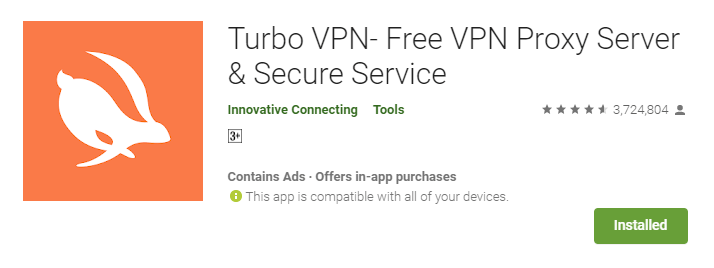The image is a horizontal rectangular screenshot of a mobile application interface for "TurboVPN-Free VPN Proxy Server and Secure Service." On the left side of the frame, there's a prominent large orange square featuring a white outline of a rabbit in motion, symbolizing speed and agility. The rabbit's front legs extend towards the left, while its back legs point to the front, creating a sense of dynamic movement.

At the top of the frame, the app's name "TurboVPN-Free VPN Proxy Server and Secure Service" is displayed in large, bold font. Below this title, in smaller green font, are the words "Innovative Connecting Tools." To the right of this line, the app's rating is shown in gray font: 4.5 stars based on 3,724,804 reviews. 

Towards the bottom of the frame, the information mentions that the app contains ads and offers in-app purchases. It also states that the app is compatible with all your devices. In the bottom right corner, there is a green button labeled "installed," indicating that the app is already downloaded on the device.